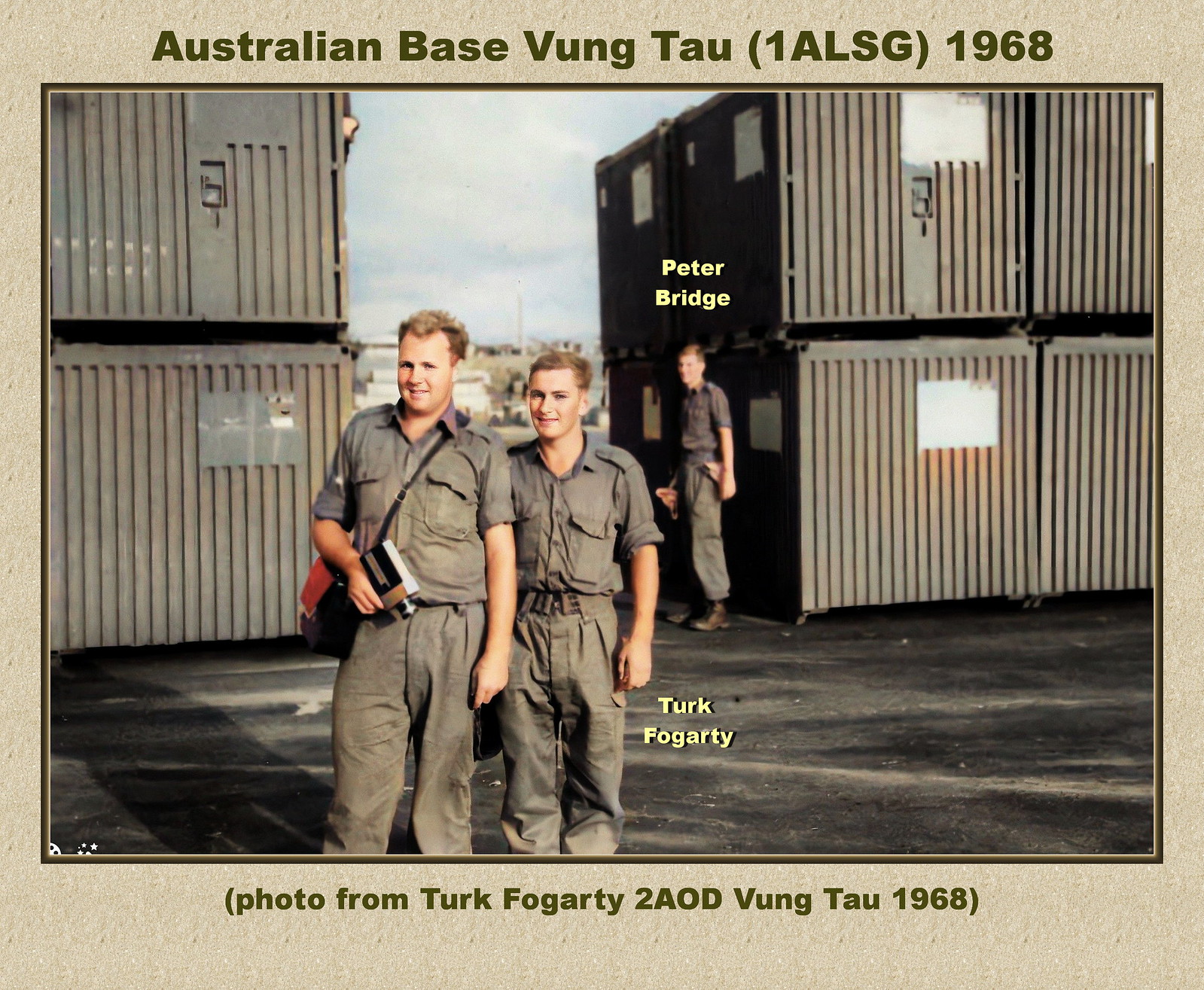This photograph, framed by a gray border, captures a scene labeled in green print at the top as "Australian Base Vung Tau (1ALSG) 1968." It depicts an outdoor daytime setting, possibly a dock or storage area, with large gray metal crates seen prominently in the background. On the left, two crates are stacked, while on the right there appear to be four crates. In the foreground, two young Caucasian men, likely in their early twenties, stand side by side, each with short blondish-brown hair, dressed in gray uniforms suggestive of military attire. The man on the left is holding an unidentified object and has a strap slung over his shoulder. To the right of the shorter man, the name "Turk Fogarty" is inscribed in yellow letters. In the background stands another man in similar attire, labeled "Peter Bridge" also in yellow text. At the bottom margin of the photo, a caption reads, "Photo from Turk Fogarty to 2AOD Vung Tau 1968."